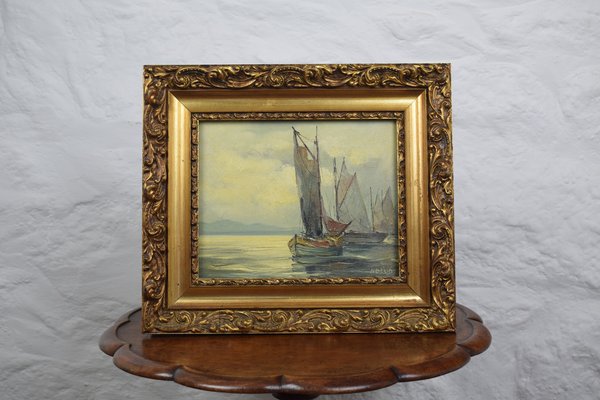The photo displays a framed painting set atop a small, round, dark wooden side table. The frame of the painting is quite elaborate, featuring a thick, large, gold-colored frame with intricate, vine-like etchings and a wavy design. Inside this is another solid gold frame, followed by a third, smaller golden frame that is once again etched with detailed patterns. The painting itself depicts a calm body of water with multiple sailboats. One boat appears to be returning to the coast, another seems to be resting in the water, and several more are visible in the distance against the horizon. The backdrop reveals mountain shapes and a sky dotted with clouds, along with the sun's reflection on the water. The image carries a subtle signature in the bottom right corner, though it is too small to decipher. The side table is placed against a white or gray wall, enhancing the visual contrast of the scene.